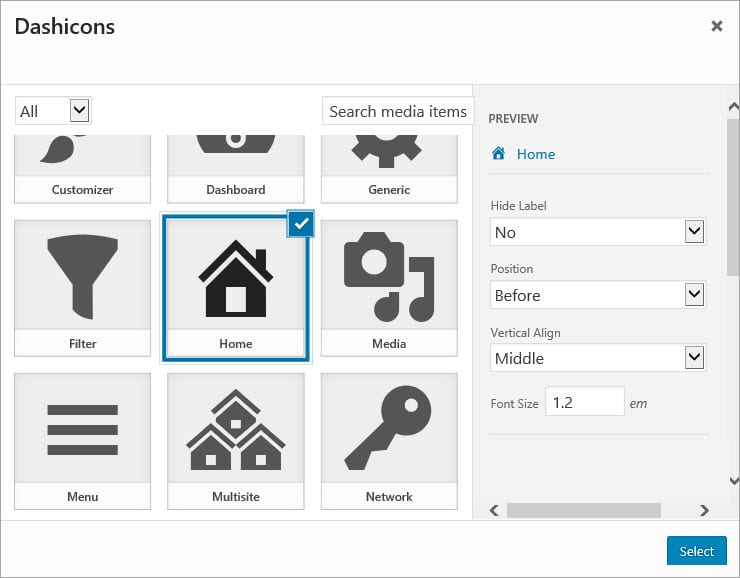In the image, a user interface is displayed against a white background. The interface includes several icons and options. At the top-left, there are 'X' icons, indicating the option to close or delete. To the right, there are categories listed: 'All,' 'Customizer,' 'Dashboard,' 'Generic,' 'Filter,' and 'Home,' with a blue square highlighting the 'Home' category. This blue square has a white checkmark inside it, indicating it is the selected option.

Additionally, there are more menu items including 'Media,' 'Menu,' 'Multi-site,' and 'Network.' Below these menu options, a gray rectangle is visible with various labels such as 'Preview,' and 'Home' which is highlighted in blue, possibly indicating another selected state. Other labels in the gray rectangle include 'Hot label,' 'Position,' 'Before,' 'Vertical,' and 'Long,' pertaining to layout or placement settings. There's also a font setting labeled 'Font Size: 1.2 EM.'

The gray rectangle features scroll bars on the right side and at the bottom, allowing for additional content to be viewed. At the bottom right of the gray rectangle, there's a blue button labeled 'Select' in white text, suggesting an action or confirmation step.